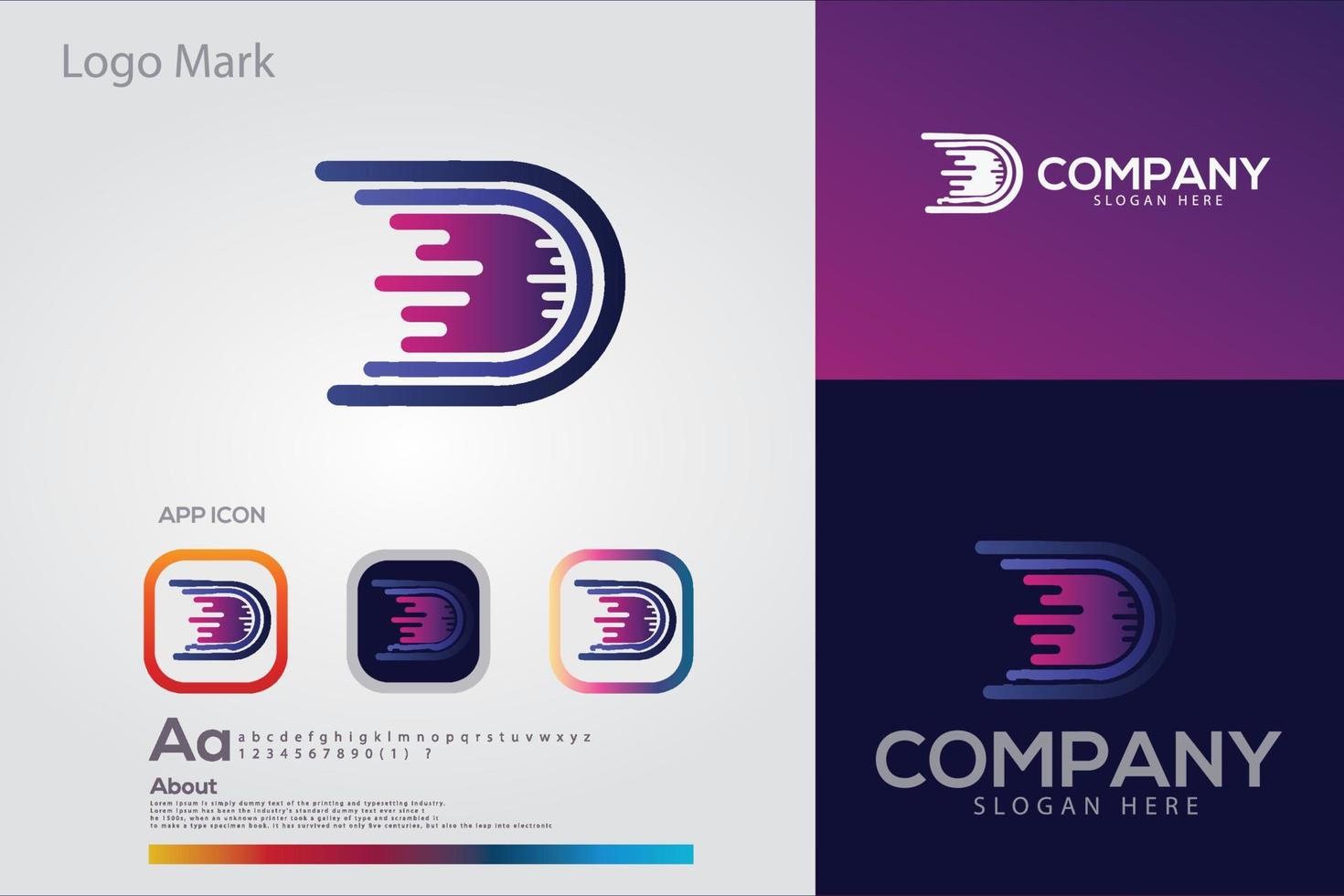The digital artwork showcases a detailed exploration of a company's logo through various adaptations and contextual presentations, using a color palette dominated by shades of magenta, purple, dark blue, and occasional touches of orange and yellow. 

On the left side of the composition, set against a gray background, the focal point is labeled "Logo Mark" and features the logo in a magenta-purple gradient transitioning to black. Below this, a section marked "App Icon" presents three app icon variations, each displaying the logo within a square: one with a plain gray background, another with a red-to-yellow gradient, and the third with a yellow, pink, and blue gradient. This section also includes placeholder text featuring a capital "A," lowercase "a," the alphabet, numbers, and a question mark.

The right side of the image is divided into two distinct areas. The upper right section features the logo in white on a purple background, accompanied by the placeholder text "Company Slogan Here." Directly below, another version of the logo is rendered in a purple and blue gradient, set against a navy background, also with the text "Company Slogan Here" in gray. Each logo variant here shares the same U-shaped design, resembling a 'U' or a 'D' without the long line, outlined in different colors to signify the brand’s versatility.

Overall, this composition reflects the branding initiative by presenting multiple interpretations and uses of the company's logo, emphasizing its adaptability across different contexts and color schemes.